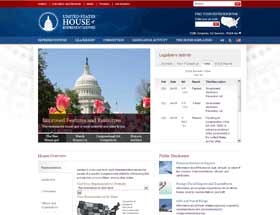The image depicts a blurry screenshot of what seems to be a government website. Across the top of the page, there is a slim red navigation bar with various headings in white text, allowing users to click through different sections of the site. On the right side of this red bar, there is a search bar for convenient access to specific information.

Beneath the red bar is a significantly thicker blue bar, approximately three or four times the thickness of the red one. On this blue bar, to the left side, there is an illustration of a building inside a circle, filled in white with minimal detail, showcasing a simplistic design featuring a pointed roof and a rounded base. Next to this, a text reads "House of." Farther to the right, positioned towards the center-right of the blue bar, there's an image of the United States map also colored in white. To the left of this map, another search bar is visible, hinting at additional navigational aids below.

Moving to the center of the page, there is a live, detailed image of a building, visibly the same as the one depicted within the blue bar’s circle, now surrounded by vibrant pink and yellow flowers, positioned on the left side. Adjacent to this live image, on the right side, there is a table containing text in black font on a white background; however, the specific content of the writing is obscured.

Beneath this section, more text is faintly visible against the website's white background. Here, another depiction of the United States map is shown, this time with several states shaded in black, gray, and white. To the right of this visual, there are numerous links, possibly leading to further information or news stories on the website, allowing users to delve deeper into its contents.